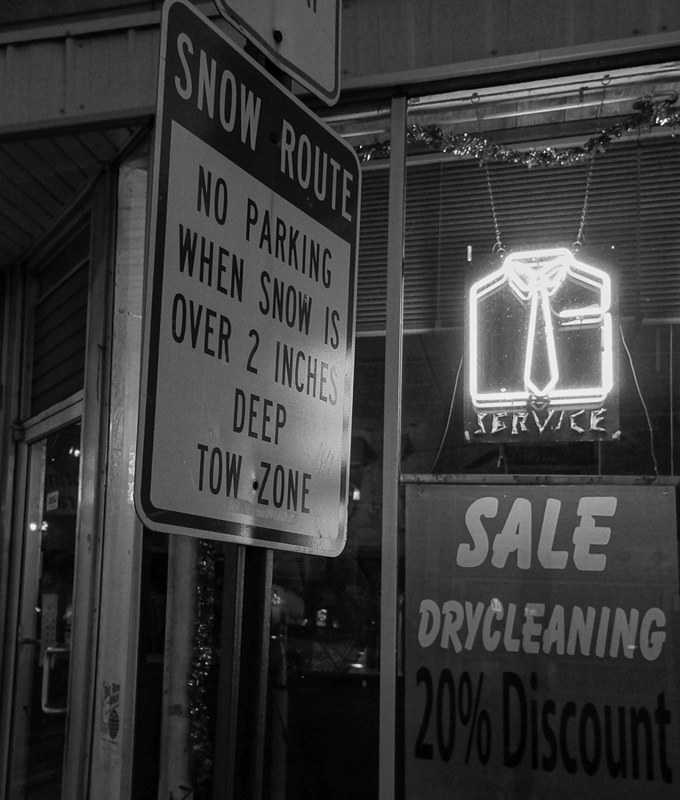This black and white photograph captures the exterior of what appears to be a dry cleaning business. Centrally prominent in the image is a square-shaped street sign attached to a metal pole, placed at a diagonal angle. The sign is segmented into two parts: the top part, against a black background with white letters, reads "SNOW ROUTE." Below it, against a white background, the text reads "No parking when snow is over two inches deep. Tow zone."

To the right of the street sign, there is a notable neon light of a shirt and tie, suggesting the business offers dry cleaning services. Below this illuminated shirt and tie, a sign reads "SERVICE." Another sign below that, in all caps white letters on a black background, announces "SALE DRY CLEANING 20% DISCOUNT."

To the left of the street sign is a door with a window likely leading into the business. Visible through the window are several shades, which are closed at the top. Despite some indistinct shapes inside, no clear people can be seen. The overall scene is predominantly in tones of black and gray, emphasizing the stark contrast characteristic of black and white photography. The image meticulously details the elements that define the storefront and its signage.